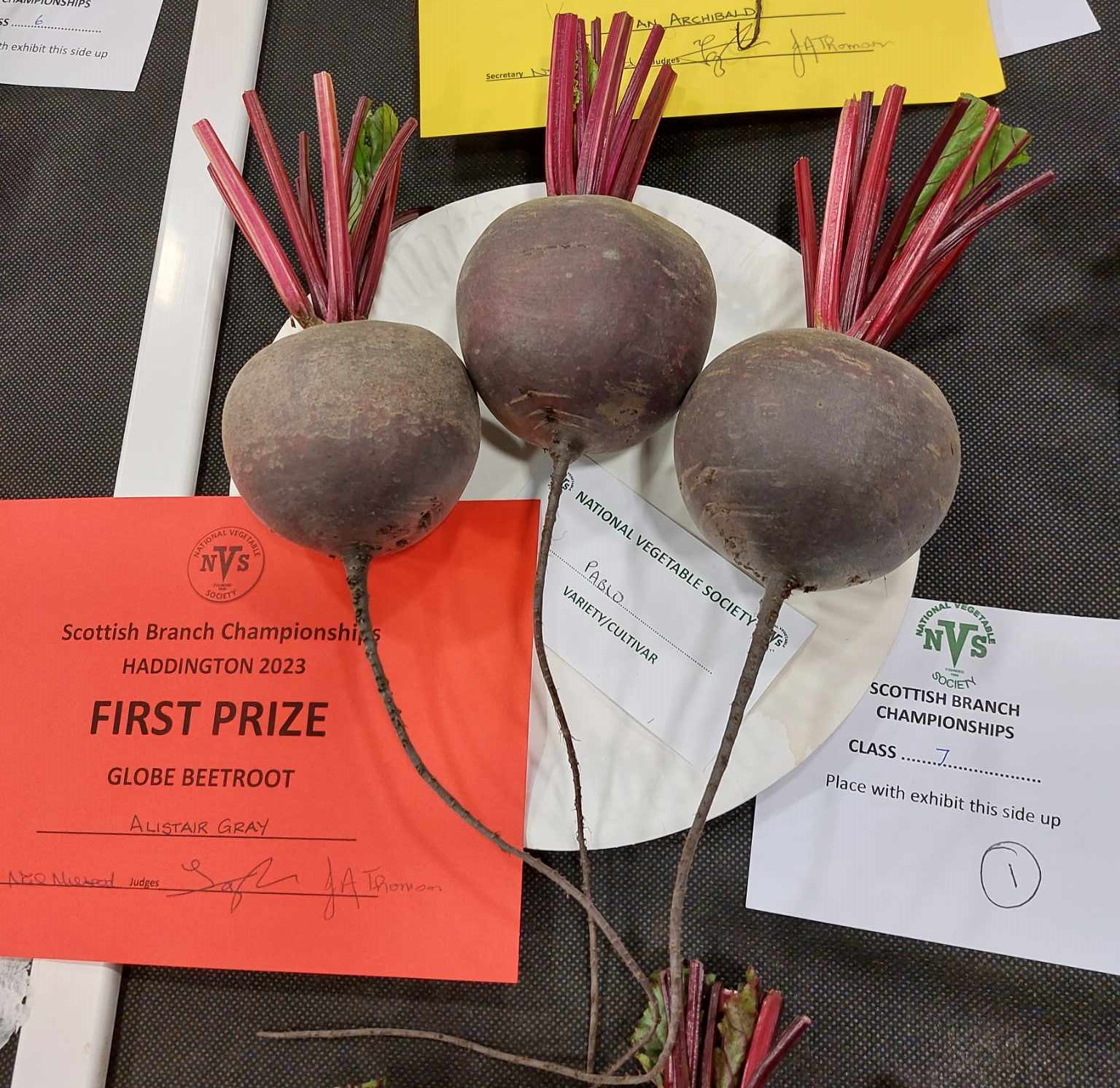The image showcases three neatly trimmed beets presented on a white paper plate, which is placed on a dark gray tablecloth. These beets were part of a competitive presentation, likely related to a county fair or an agricultural contest. An orange slip of paper beside the plate indicates that they were entered in the National Vegetable Society Scottish Branch Championships, Haddington 2023, under Class Seven for globe beetroot. The beets secured the first prize, with the entry listed under the name Alistair Gray.